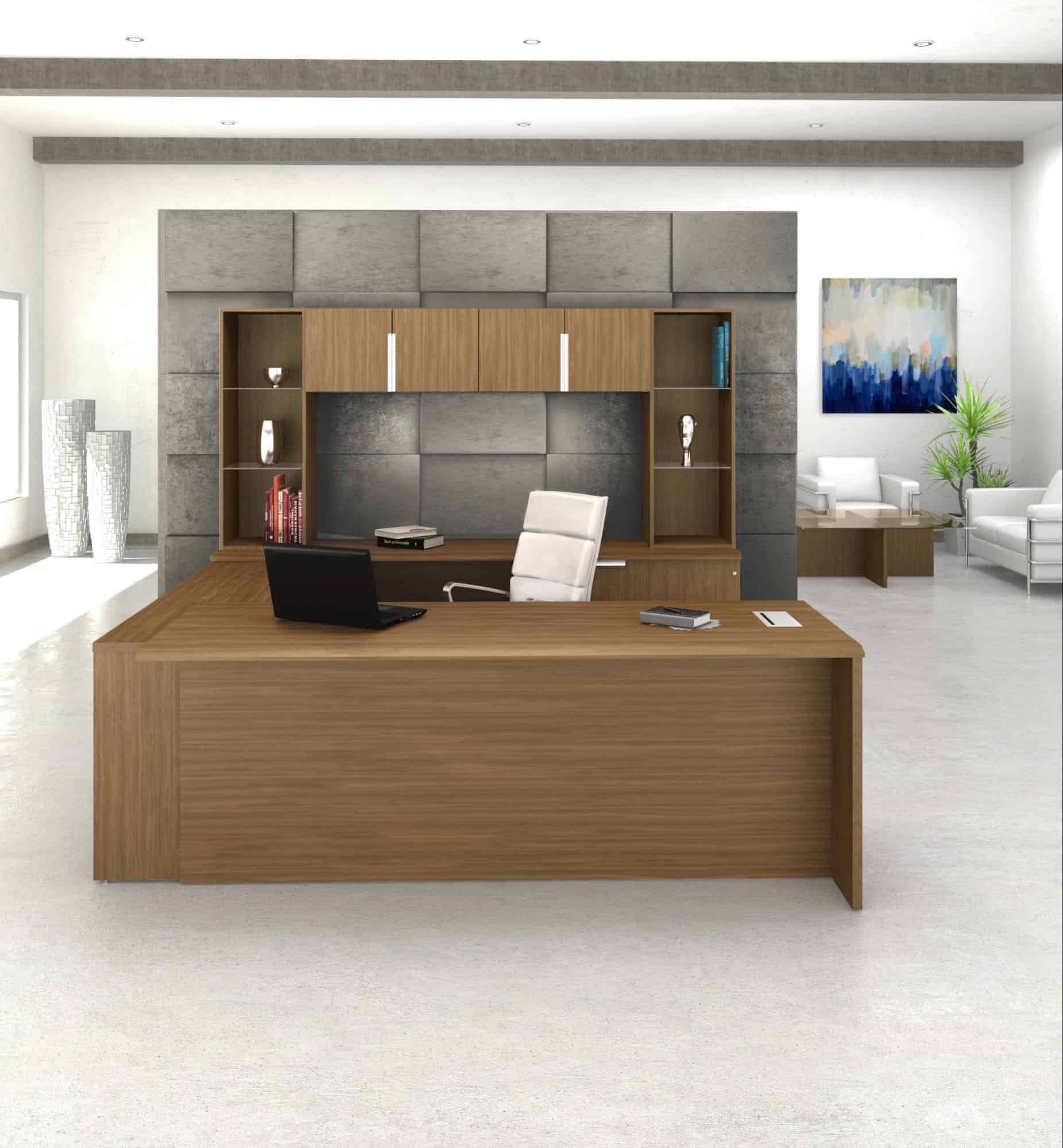The image depicts a modern office space featuring a white office chair situated behind a large U-shaped wooden desk. Atop the desk lies a black laptop, along with a piece of paper and a book towards the front. The desk's backdrop includes a bookshelf filled with various books, two glasses, a trophy, and additional storage cabinets. The office room's walls are white, with a brick accent wall partially visible behind the shelves. A vibrant, abstract blue painting adorns the back wall, adding a splash of color. A green bush is nestled in the left corner near the window, while to the right, a small love seat and a short wooden and glass-topped table create a cozy waiting area. The overall atmosphere is bright, clean, and organized, incorporating a serene color palette of light Wedgewood, gray, and blue tones.